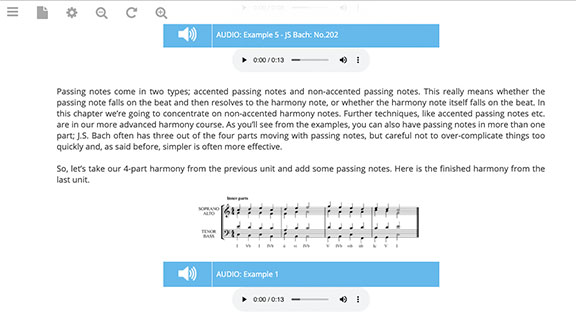This screenshot shows a section of a monochromatic website dedicated to audio samples and harmonies, featuring a significant amount of text describing various aspects of musical harmonization. The text is somewhat small and dense, making it challenging to read without visual aids. The page includes several 13-second audio recordings, highlighted in blue to distinguish them from the otherwise black and white interface. These audio clips appear to be samples or examples provided for users seeking advice or feedback on their harmonic techniques. The overall design of the website is quite simplistic, focusing on functionality rather than aesthetic appeal.